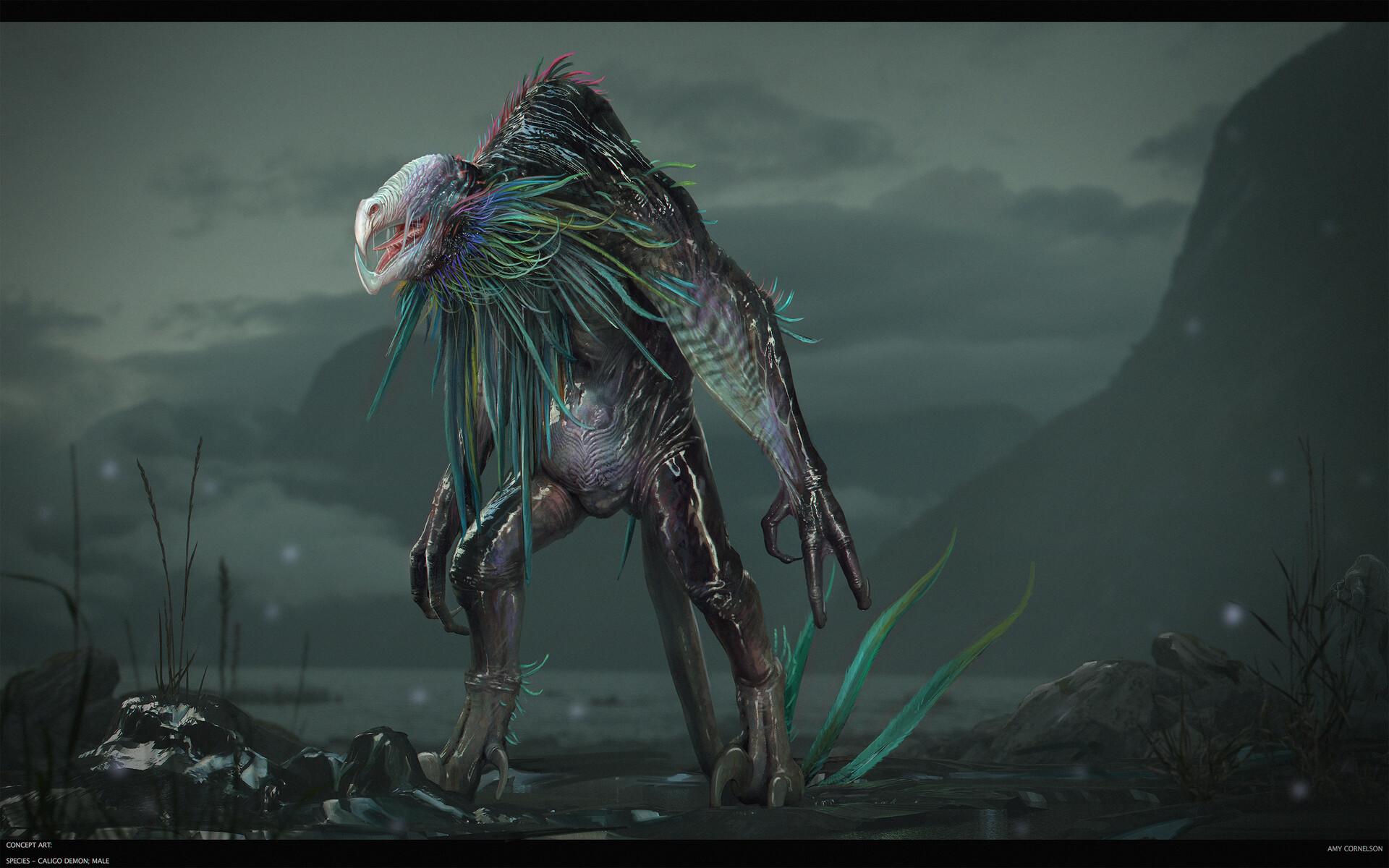In a vibrant and mystical landscape featuring blurred, greenish-gray mountains and ominous clouds, a monstrous, fantastical creature towers in the foreground. The creature appears as an amalgamation of various animals and possibly plants, bearing characteristics of insects, squids, lizards, and tropical birds. Its formidable three-clawed feet resemble those of a Tyrannosaurus rex, anchoring its tall and imposing frame. The body transitions from dark purple to a translucent black, shimmering with shades of silver and purple, leading up to a massive, humped back adorned with fur-like, feathery appendages.

Brightly colored scales or feathers in hues of purple, blue, multiple shades of green, red, and rose cascade around its neck and down its back, almost reaching the ground. These radiant feathers also adorn the creature’s elbows and heels. The head, reminiscent of a vulture, is a striking combination of shiny silver and purple, with a prominent red tongue protruding from its beak-like mouth. One can't discern any eyes, but a nostril is visible, adding to its eerie appearance.

The creature's disproportionately large three-fingered claws extend from ginormous forearms, and these black, spiky fingers contribute to its menacing demeanor. In this otherworldly setting, the viewer looks up at the colossal, evil-looking being, which exudes an aura of danger and mysticism, amplified by the dim, rocky foreground scattered with twigs and a dark, dirt terrain.